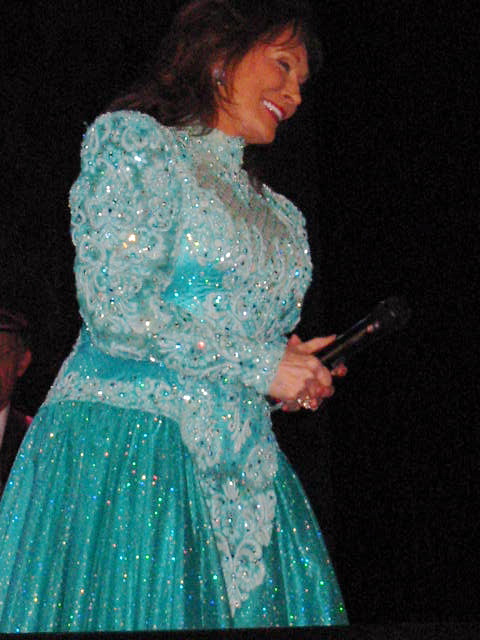The photograph captures a vibrant stage event with a black background. At the center, a woman wearing a shimmering blue gown adorned with intricate patterns and embellishments holds a black microphone with both hands. Her brown, shoulder-length hair frames her face as she smiles warmly, her gaze directed downward. She wears pink nail polish, a ring, and a visible earring. The image is taken from a low, side angle, emphasizing the sparkle of her dress. In the background, to the right, another person can be seen standing, though their face and details are indistinguishable.